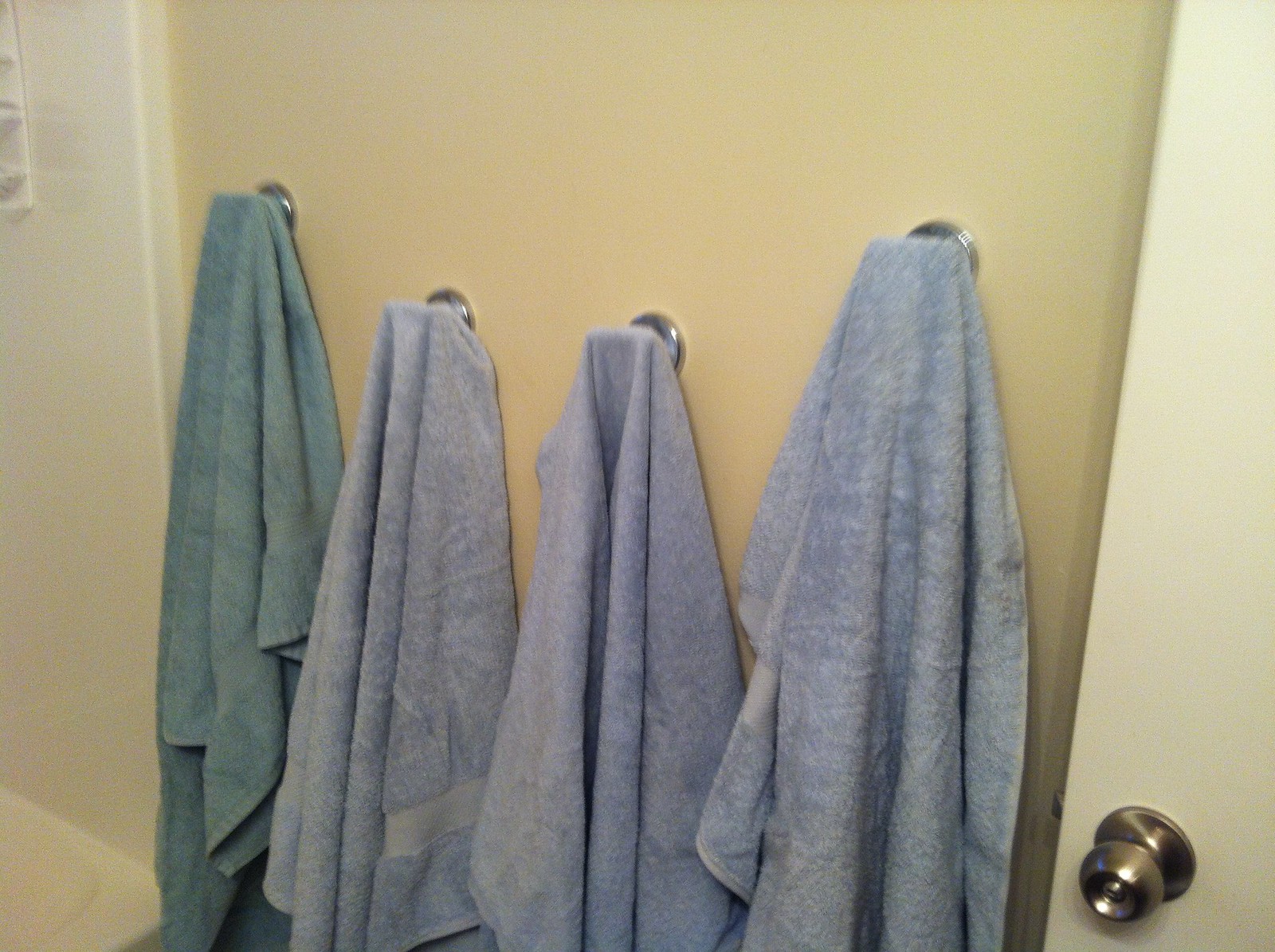This photograph captures a detailed scene within a bathroom. To the left, we can see a corner of a white tub and part of a plain white wall. There's also a small shelving unit or a soap dish visible on this wall. The main focal point of the image is the four towels hanging on silver hooks which are partially obscured by the towels themselves. Three of the towels are a light, muted lavender color, while one is a light teal color. All the towels appear plush and absorbent, indicative of good quality, but they are somewhat dirty and well-used. They are hanging rather low on a wall that shifts from an off-white to a pastel yellow hue, maybe even a light beige, which adds a warm tone to the bathroom. On the far right, the image captures a glimpse of an open door with a silver knob. The door is a whiter shade compared to the wall. The overall ambiance suggests a well-used but functional bathroom shared by multiple people, with a standard, builder-grade aesthetic.